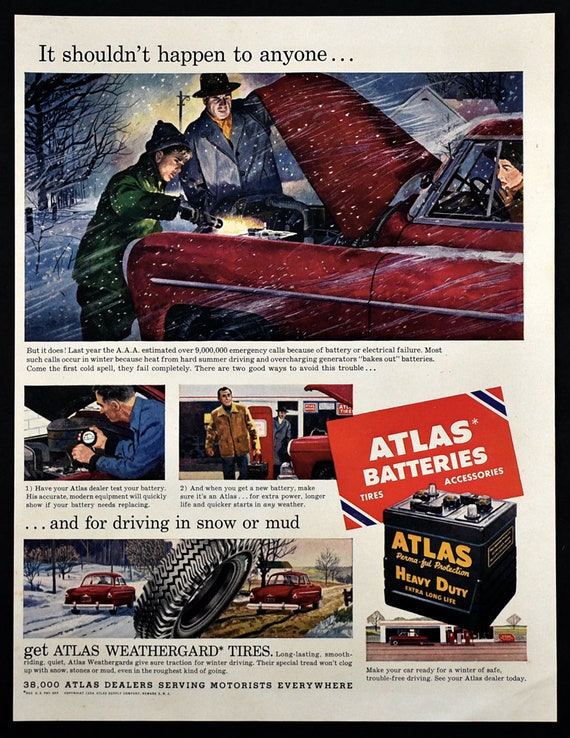The image is a full-page vintage advertisement for Atlas Batteries, Tires, and Accessories, framed in black. At the top, the ad features the headline "It shouldn't happen to anyone..." followed by an illustrated scene of a snow-covered, red 1950s car with its hood up. A man and a young boy holding a flashlight examine the car's engine while a woman sits inside the car. Below the main illustration, the text details the common issues faced by drivers in winter, stating that "Last year, AAA estimated over 9 million emergency calls because of battery or electrical failures."

Additional smaller images accompany the main scene: one shows a mechanic at work, and another vignette is difficult to discern but seems related to car troubles. Further down, there's a depiction of a tire transitioning between snow and mud, emphasizing the challenges of winter driving. The ad advocates for Atlas Weather Guard Tires, and to the right, there's a visual of a black battery labeled "Atlas Heavy-Duty" with a red placard above it reading "Atlas Batteries." Text surrounding these images encourages consumers to trust Atlas for reliable batteries and tires to avoid winter driving mishaps.